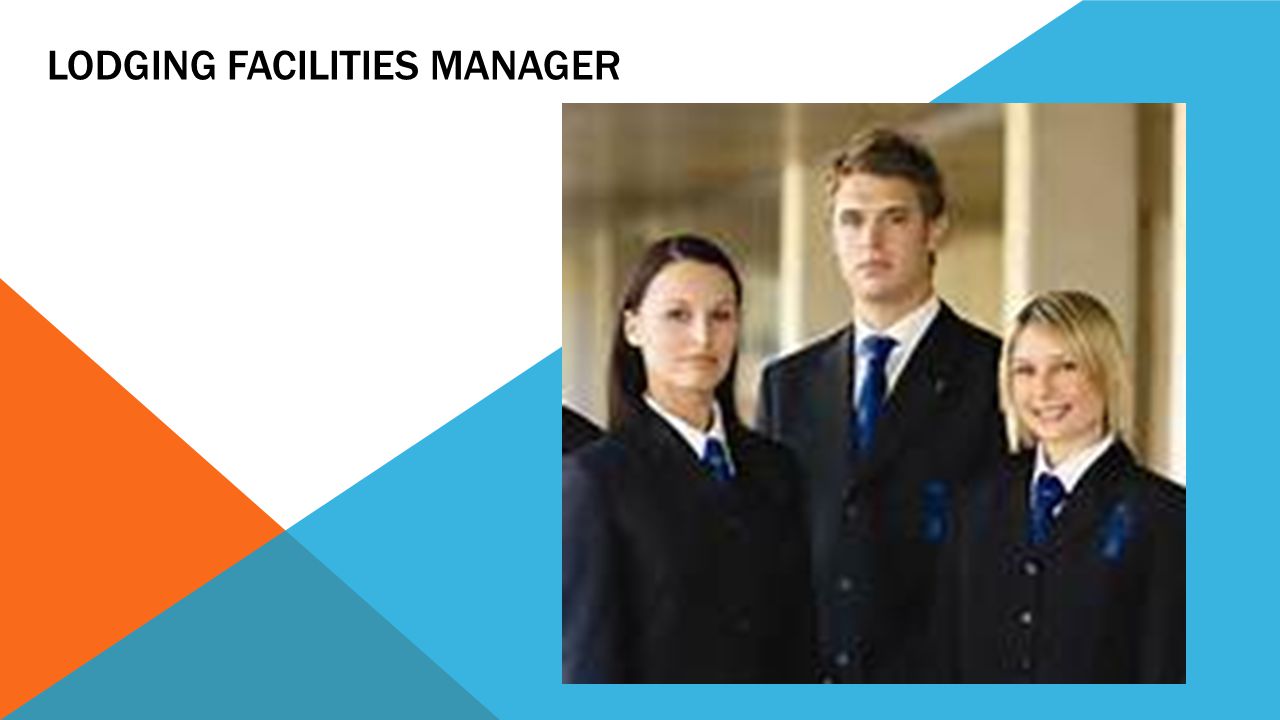The image showcases a PowerPoint slide with a colorful, multi-hued background in shades of white, orange, and blue. In the upper left corner, the text "Lodging Facilities Manager" is prominently displayed in black. The focal point is a square photograph on the right side, featuring three formally dressed individuals. Their attire is uniform, consisting of black suit jackets, white collared shirts, and blue ties. On the far right stands a blonde-haired woman with a blue ribbon pinned to her jacket. In the center is a tall man with short brown hair, flanked by a brown-haired woman on the left. All three individuals are in their twenties, standing with good posture against a blurred background that includes white pillars. The overall image quality is noted to be poor.